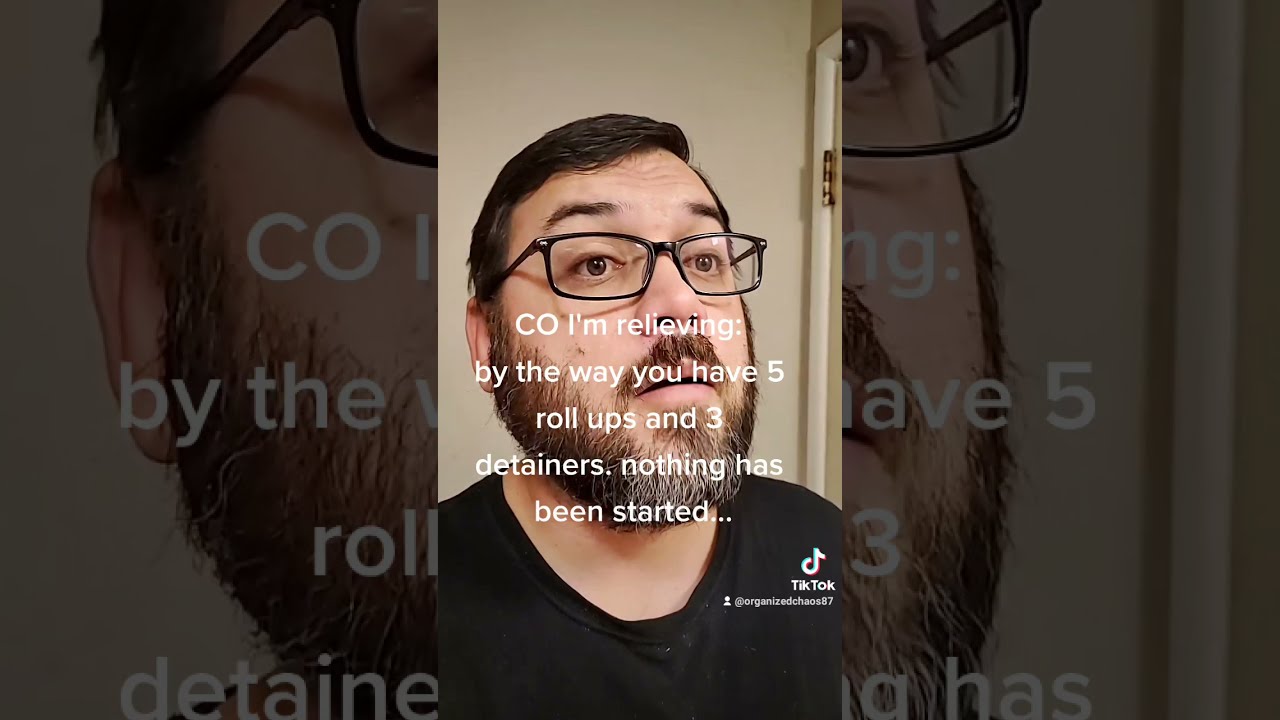This image from TikTok features a middle-aged white man with short brown hair, styled and parted to the left, and a brown beard that is slightly gray at the tips. He wears square, boxy glasses and a black t-shirt, and his face is shown from the chest up. The man is looking up and to his left, with his lips slightly open and eyebrows raised. Superimposed over his face in white text is the caption: "CEO, I'm relieving: By the way, you have five roll-ups and three detainers. Nothing has been started..." Additionally, a TikTok logo is visible on his shoulder with his handle, "organized_chaos87," below it. The background features a partial view of what seems to be a room, possibly a bathroom, indicated by a door hinge. The sides of the image have filler graphics, displaying zoomed-in, less focused close-ups of his face and the caption, set against an opaque black background, to fit the vertical image into a landscape format.